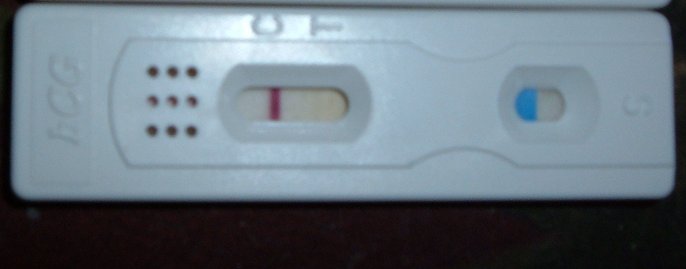A white or slightly off-white rectangular object, likely a pregnancy test, is placed horizontally on a dark brown, wood-toned surface. The left side of the device features the acronym "HCG," indicating its purpose as an HCG (human chorionic gonadotropin) test, commonly used for pregnancy detection. On the far right, there's a small section marked with an "S," and adjacent to it is a tiny window with a blue component, contrasted by an empty or clear section beside it. The middle of the test has a larger, oblong window, which is at least twice the size of the smaller one. This window has a red line and a cream or off-white background. Above the window, are two indistinct markings. The oblong window is flanked by nine small holes, whose purpose is unclear.